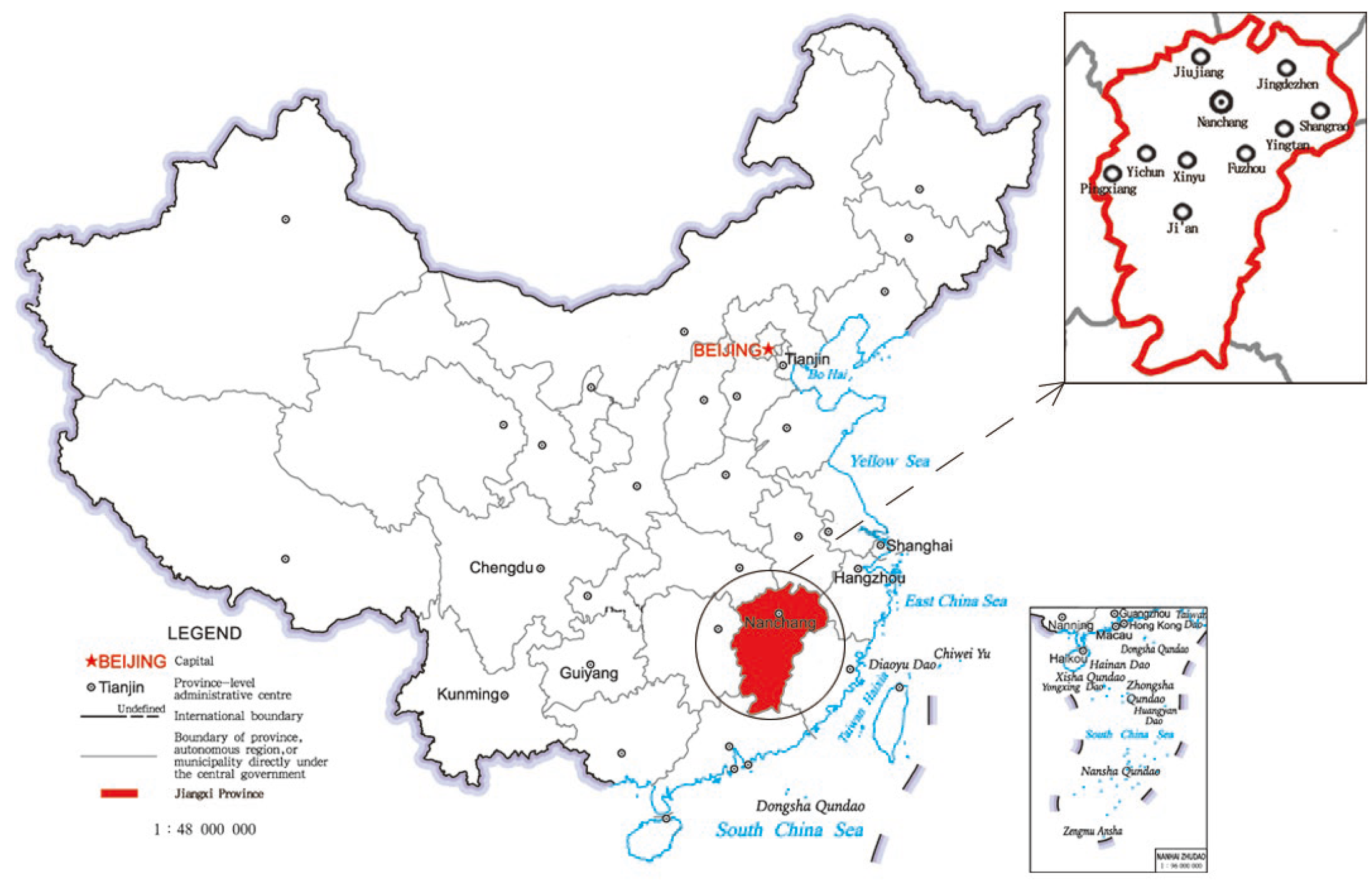This image features a detailed map of China, primarily in black and white with an array of labeled geographical and political elements. The map covers the majority of China, with individual provinces clearly marked and large cities identified. The map legend, located in the bottom left corner, uses a red star to denote Beijing, the capital, labeled as such in black text. It also includes a gray circle representing major cities, with markers for province-level administrative centers and various boundaries such as international boundaries and provincial borders.

A prominent feature of the map is a close-up inset of Jiangxi province, located in the top right corner, connected by a black dotted arrow. The inset highlights cities like Chujing, Jingyishen, Nanchang, Shengrao, Yingtan, Fushu, Xinyu, Yichun, Pingxiang, and Jian.

The map also names several significant bodies of water along the eastern coastline, including the Bohai to the north, followed by the Yellow Sea, the East China Sea, and the South China Sea moving southwards. Additionally, Taiwan is labeled further east.

This map emphasizes the major urban areas and maritime boundaries, providing a comprehensive overview of China's geographical landscape and administrative divisions.